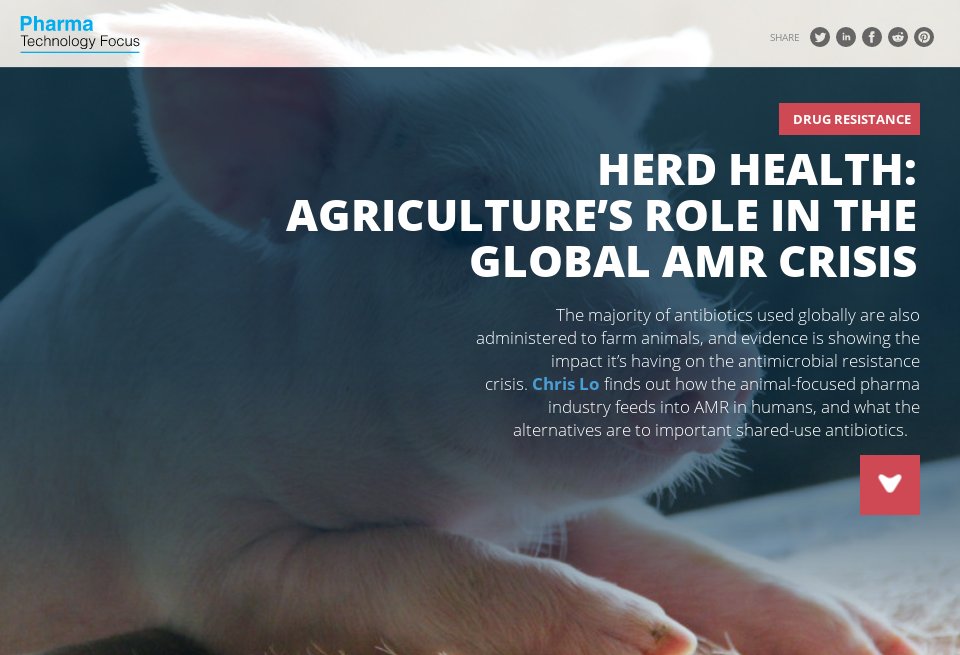This detailed caption describes an image featured on a webpage produced by Pharma Technology Focus. The top-left corner prominently displays the Pharma Technology Focus logo. The central visual is a partially shaded image of an adorable, very young pink pig with distinctive large pink ears. The pig's image is layered under a black-gray shading effect, adding depth and focus to the image.

At the top of the image, a red box contains the words "Drug Resistance" in bold white font. Below this, in very large white letters, the title reads: "Herd Health: Agriculture's Role in the Global AMR Crisis." Following the title, a paragraph begins, explaining the content: "The majority of antibiotics used globally are also administered to farm animals and evidence is showing the impact it's having on the antimicrobial resistance crisis. Chris Low finds out how the animal-focused pharma industries feed into the AMR in humans and what the alternatives are to important shared-use antibiotics."

Beneath the paragraph is a red square with a white heart symbol, indicating the importance of the topic and likely providing an option to engage further. Social media icons for Twitter, Facebook, and three additional platforms are displayed at the top right, offering options to share the content. This well-designed webpage invites readers to explore the critical issue of antimicrobial resistance (AMR) in the context of agriculture and animal health.